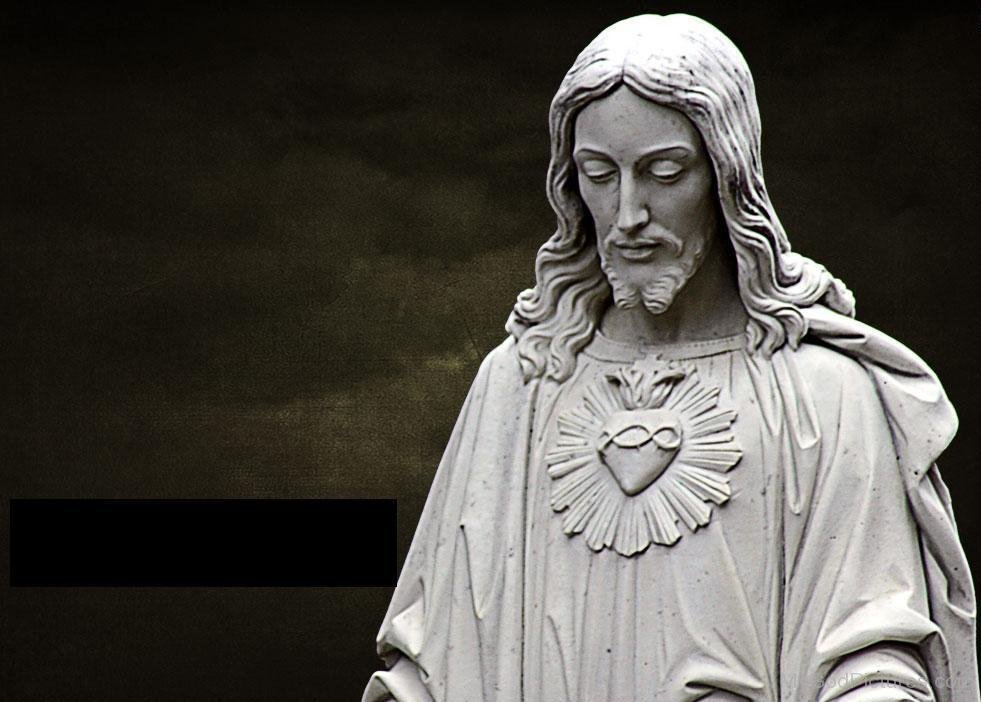This photograph features a detailed view of the Sacred Heart statue of Jesus, focusing on the area from the elbows upward. The statue, often associated with Catholic iconography, portrays Jesus with distinctive features: a slight mustache, a modest beard, and long, flowing hair. His face, characterized by slim features, holds a contemplative downward gaze.

Adorning his chest is the iconic Sacred Heart, intricately designed with a cross and a crisscross pattern resembling the ichthys, or fish symbol, encircling it. Above the heart, a star-shaped medallion adds to the statue's rich detailing. Jesus is depicted wearing a flowing garment with a cape-like drape in the background, adding to the statue’s majestic aura. The statue itself is rendered in an off-white or very light gray hue.

The background of the image is predominantly dark with subtle variations, creating an edited, almost mysterious effect. Notably, a black bar appears in the lower left corner, suggesting something has been obscured or blotted out. This enigmatic backdrop further emphasizes the serene and solemn expression of the Sacred Heart statue.